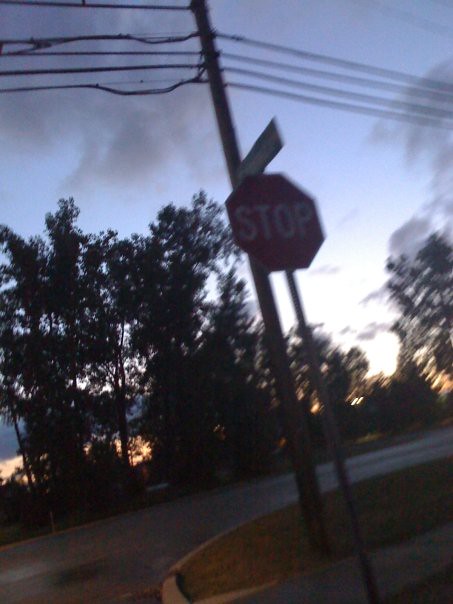An outdoor image taken at dusk or nighttime, capturing a slightly motion-blurred street corner scene. The sky transitions from light to dark blue with tinges of gray and scattered, tinted gray clouds suggesting possible rain. The foreground prominently features a stop sign at the center, slightly blurred due to movement, with an unreadable street sign above it. Behind the stop sign, a tall telephone pole with multiple wires extends upward, centralized in the photo. Below, a sidewalk runs through a concrete area separating it from a strip of dry grass between the curb and the sidewalk. Across the street, tall trees, silhouetted against an orange-tinged horizon, complete the scene's backdrop.